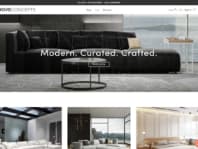This image captures a snapshot of a contemporary website showcasing modern furniture. Prominently displayed at the top, bold text reads "Modern. Curated. Crafted." each word separated by a period, emphasizing the brand's focus on meticulously selected and designed pieces. The central visual element is a sleek, elongated leather couch positioned in an elegantly modern space accentuated by large windows, contributing to an open and airy ambiance. Above the main image of the couch, there's a large black rectangular banner stretching across the width of the website. Beneath this, a larger white rectangular section spans the screen, doubling the height of the black banner. As you scroll further, the lower section features a series of images that, despite their small size, offer glimpses of various stylish furnishings. These include not just the highlighted couch but also ceiling lights, cupboards, and other beautiful pieces, each contributing to the overall modern aesthetic of the interior scene.